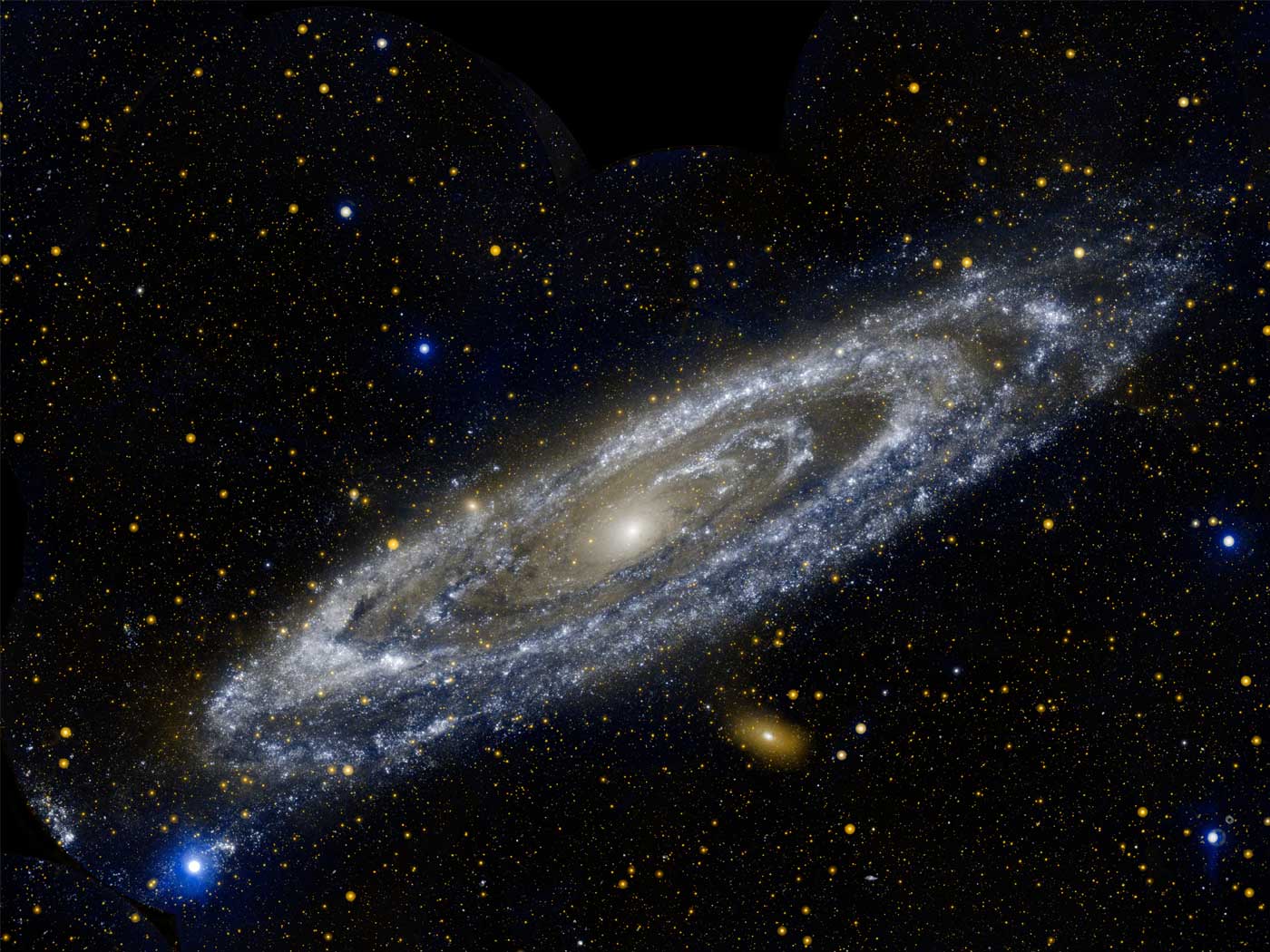This illustration showcases a large spiral galaxy, prominently positioned diagonally from the bottom left to the top right of the image. The galaxy’s core features a notably bright white star. The spiral arms emanate in a milky, silver cloud-like formation, interspersed with countless stars. Surrounding the galaxy, in the vast, black expanse of space, are numerous stars of varying sizes and colors: predominantly white and yellow, with around seven or eight blue stars scattered throughout. Some celestial bodies are larger and appear as glowing balls in hues of yellow and blue, while others are mere specks or dots. Additionally, the image hints at the presence of potentially other galaxies in the distance, suggested by the shape and light filtering of some larger star-like objects.